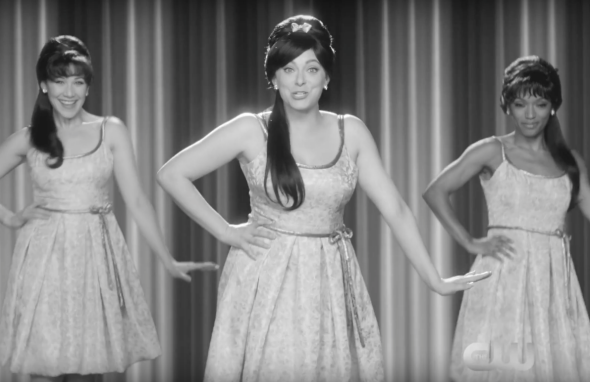This vintage black-and-white photograph, likely from the 1950s or 1960s, showcases three poised women standing on a stage adorned with a curtain backdrop, featuring alternating bright and dark vertical stripes. Each woman is dressed identically in a white scoop-neck dress that cinches at the waist with a cloth belt and ends right at the knees. Their hairstyles are similarly styled, with hair partially in buns, parted with straight bangs, and a ponytail draping over the shoulder — the women on the left and center have their ponytails over the right shoulder, while the one on the right has hers over the left shoulder. The women, grouped with two white women on the left and a black woman on the right, all strike the same “teapot” pose, with their right hands on their hips and left arms extended outward, palms down and slightly bent at the elbows, possibly suggesting they are part of a coordinated singing or dancing group. Their synchronized pose and attire, paired with the stage setting, vividly evoke the charm and elegance typical of mid-20th century performance ensembles.